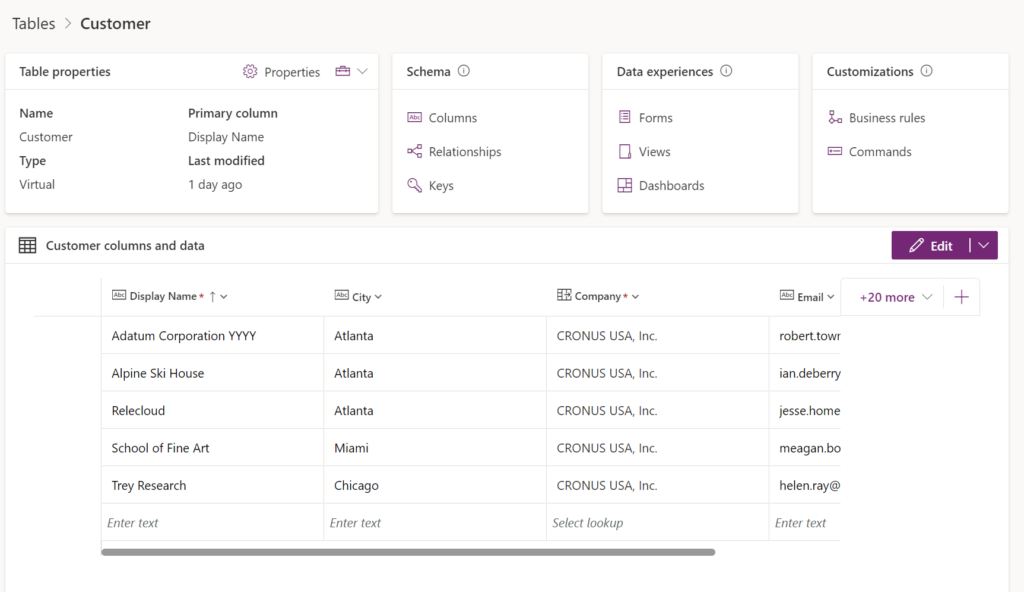The image features a light gray background with organizational elements related to data tables and customer properties. At the top of the image, the text "Tables > Customers" is prominently displayed, indicating navigation through data structures. Below this, a white box titled "Table Properties" is seen. In the top right corner of this box, an icon resembling a gear and labeled "Property" indicates settings options, with a corresponding drop-down menu.

On the left side of the box, textual details mention "Name: Customer," "Type: Virtual," and information on the right side states "Primary Column: Display Name," followed by "Last Modified: One day ago." Additionally, a smaller section titled "Schema" contains subsections for "Columns," "Relationships," and "Keys." Adjacent to this, labeled "Data Experiences," is another section with "Forms," "Views," and "Dashboards."

To the far right, there's another box labeled "Customization," which subdivides into "Business Rules" and "Commands." At the bottom of the image, a larger box titled "Customer Columns and Data" is displayed, indicating a detailed overview of customer-specific data. On the right side of this larger box, a purple box features a pencil icon accompanied by a drop-down menu labeled "Edit," suggesting options for modifying the data.

Overall, the image is a comprehensive screenshot of a data management interface, detailing various attributes and settings for handling customer data tables.